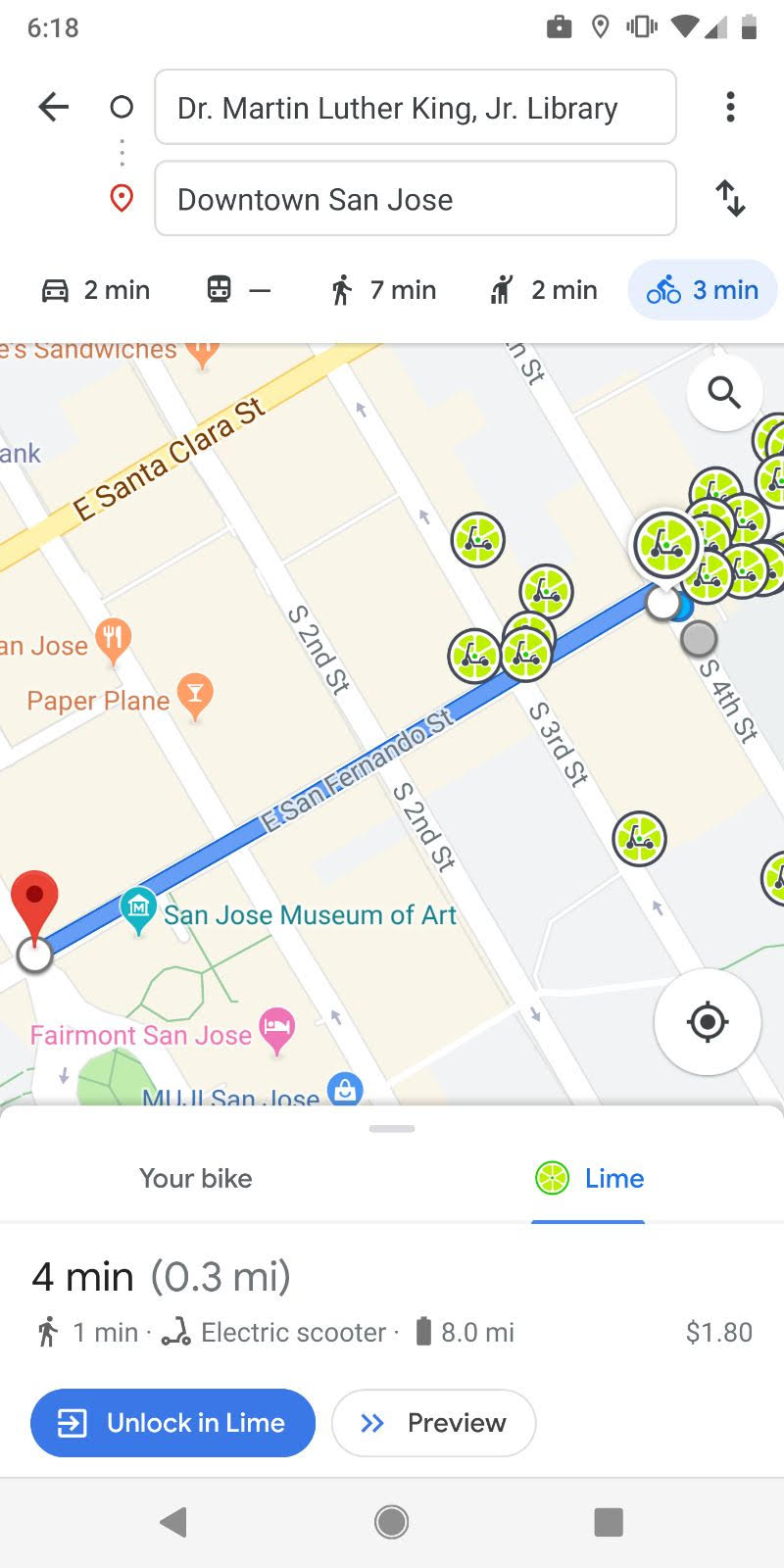A screenshot displaying a detailed user interface with various icons and text in grayscale, red, blue, teal, pink, and lime-green accents. 

At the top of the image, the status bar shows a timestamp of 6:18, accompanied by common icons: a shopping bag, a location pin, a cell phone, a Wi-Fi symbol, and a battery indicator, all in gray. Below this, there's a gray back arrow and a circle, followed by two input fields. The first input box reads "Dr. Martin Luther King Jr. Library" in gray with an ellipsis next to it. Below, "Downtown San Jose" is displayed in gray with a red location pin beside it. Adjacent to these inputs are gray up and down arrows.

Further down, the interface displays travel time options: a car icon with "2 min", a bus icon with "7 min", a walking person icon with "2 min", and a cycling person icon with "3 min" in blue. The main section of the image shows a Google Street View map with streets labeled "East Santa Clara Street," "San Jose Museum of Art," and "Fairmont San Jose." Various fonts in pink, teal, and blue are used to label points of interest. There are numerous green-background scooter icons displayed. 

A white circle with a gray bullseye icon is visible below this, adjacent to text reading "Your bike" in gray and "lime" in blue, accompanied by the Lime logo. It indicates that the electric scooter travel time is "4 min (0.3 mi)" with a walking person icon for "1 min," an electric scooter icon, "8 miles" with a battery icon, and "$1.80".

Near the bottom, a blue and white button labeled "Unlock" and "lime" is featured, with another button reading "Preview" in black and blue, followed by a gray menu tab including a back button, a circle, and a square.